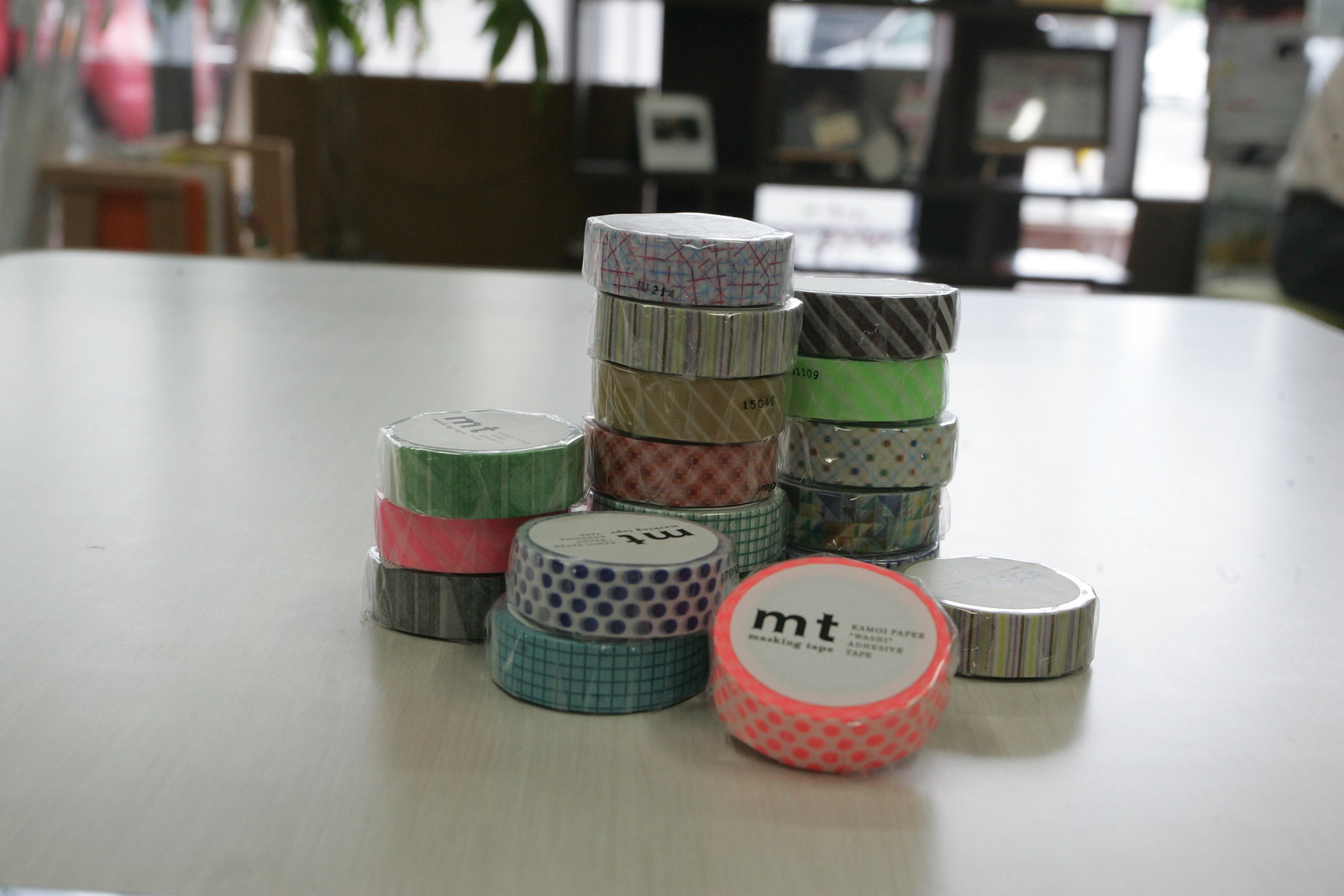This close-up photograph captures an array of new masking tapes, prominently marked with the brand name "MT." These rolls are varied in their designs—featuring a mix of vibrant patterns such as pink and white stripes, blue polka dots, black and gray stripes, green solids, and multicolored checks. Each roll is wrapped in plastic, suggesting they are brand new. The tapes are arranged in various stacks, with some reaching six or seven rolls high, while others are grouped in smaller piles or lie independently. They rest on a light-colored wooden table. In the blurred background, one can discern a room setting that includes leafy house plants, some framed photos on a shelf, and a door alongside a chair pulled up against another table, giving the scene a cozy, domestic atmosphere.